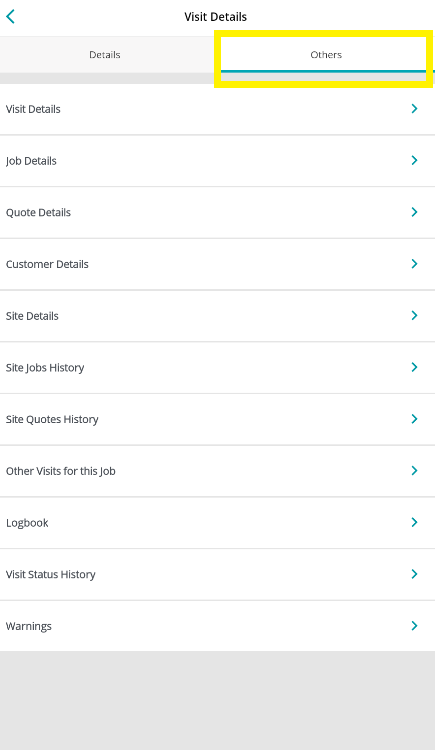The image captures a screenshot from a cell phone, showcasing a detailed and organized interface screen, specified for "Visit Details." At the top, the words "Visit Details" provide a clear header, accompanied by two tabs: "Details" on the left and "Others" on the right. Notably, the "Others" tab is highlighted with a yellow rectangular outline, drawing attention to it. Directly below this, a blue line underscores the area.

On the left side of the screen, a vertical list categorizes relevant information. Adjacent to each category on the right side of the screen, right-pointing arrows are neatly aligned within their own rectangles, suggesting expandable options. The various categories listed include:

1. Job Details
2. Quote Details
3. Customer Details
4. Site Details
5. Site Jobs History
6. Site Quotes History
7. Other Visits for this Job
8. Log Book
9. Visit Status History
10. Warnings

At the bottom of the interface, there is a light gray rectangular area that remains unused, contributing to the structured design of the screen. Each section is separated by faint gray lines, ensuring a clean and readable layout.